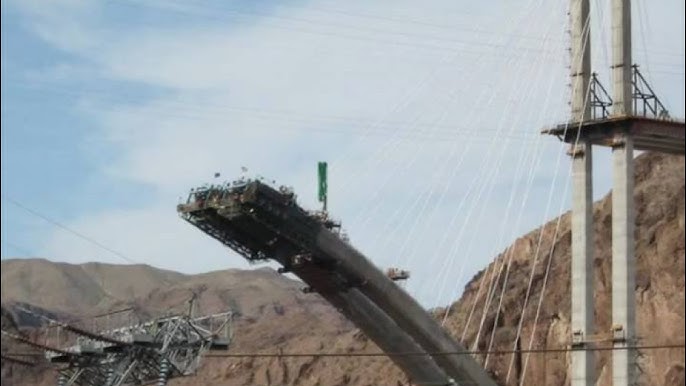The photograph depicts an outdoor scene of a bridge under construction, spanning over a rugged canyon. The central portion of the bridge is conspicuously missing, indicating that it is either being constructed or repaired. Suspended by a complex network of strings and pulleys, the middle segment of the bridge appears to be in the process of being lifted into place. The backdrop features a blue sky lightly scattered with clouds, while the foreground shows power lines and tall support towers. Dominating the lower half of the image, the canyon is composed of brown rock formations, embodying the colors gray, whitish-gray, and brown. A notable detail in the middle of the frame is a white flag or marking, contrasting with the overall construction scene. A secondary structure also under construction can be seen below the bridge. This detailed composition highlights the intricacy and scale of the engineering project set against mountainous terrain.